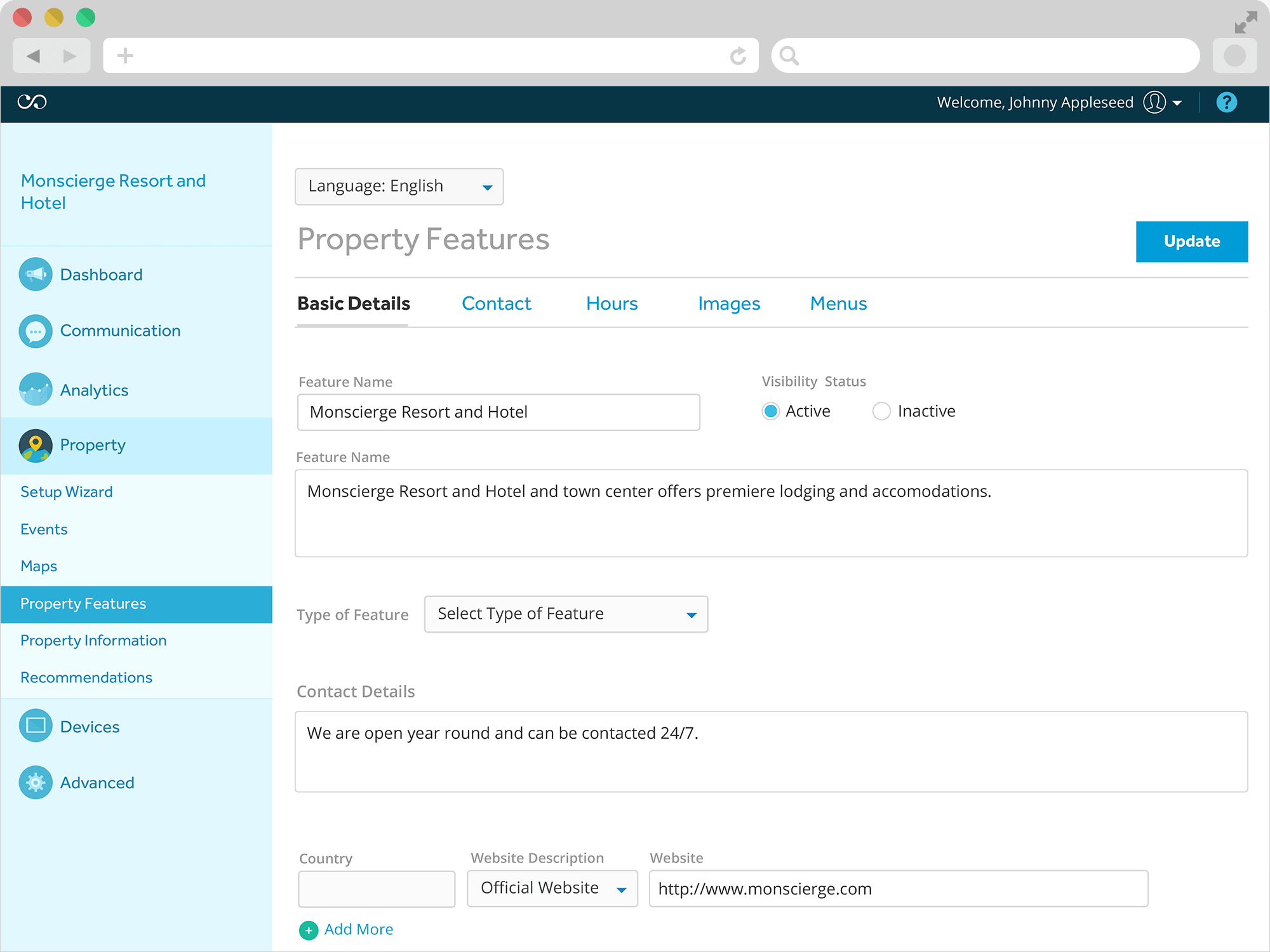This is a screenshot of the settings section on Mossier’s Resort and Hotel’s website interface. At the top, there is a dark blue bar displaying a welcome message to the user "Johnny Appleseed," accompanied by an avatar. This appears to be a sample user profile since "Johnny Appleseed" is a placeholder name commonly used for demonstrations.

On the left side of the screen, the sidebar prominently displays the title "Mossier's Resort and Hotel" and features several navigation links: Dashboard, Communication, Analytics, Property (which is currently selected), Devices, and Advanced. Under the "Property" category, there are additional options including Setup Wizard, Events, Maps, Property Features, Property Information, and Recommendations. The selected option is "Property Features."

On the main section to the right, featuring a white background, there is a language selection drop-down menu set to English. The header indicates "Property Features" with a clickable update link. Beneath that, there are links named Basic Details, Contact, Hours, Images, and Menus.

The "Property Features" section includes fields like "Feature Name," which is set to "Mossier's Resort and Hotel." The visibility status is marked as active. It also highlights that "Mossier’s Resort and Hotel and Town Center offers premier lodging and accommodations." There is a drop-down menu to select the type of feature, followed by contact details stating the property is open year-round and provides 24/7 support. Additional fields include Country, Website Description, and Website URL for users to input the resort's online address.